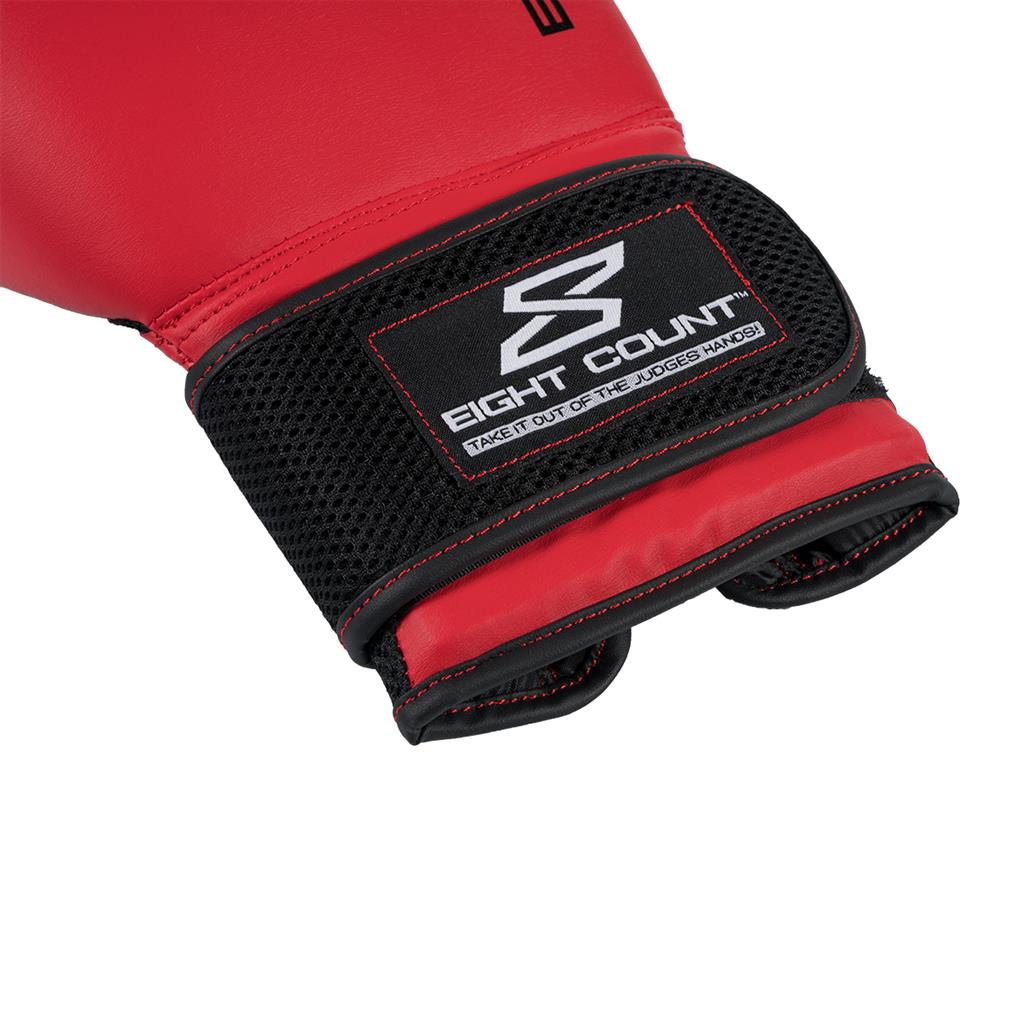This image features the bottom half of a red boxing glove prominently positioned from the middle portion of the image extending to the upper left corner. The glove's design includes a black velcro strap around the wrist area, bordered with red stitching. Attached to this strap is a black patch with a bold, angular white number '8' outlined in black. Below the number, the phrase "eight count" is displayed in white text with the tagline "take it out of the judge's hands" written in black text on a white background, seamlessly integrated into the wristband area. The glove's red leather-like texture and meticulous red thread detailing add to its striking appearance, while the white background of the image accentuates these features.